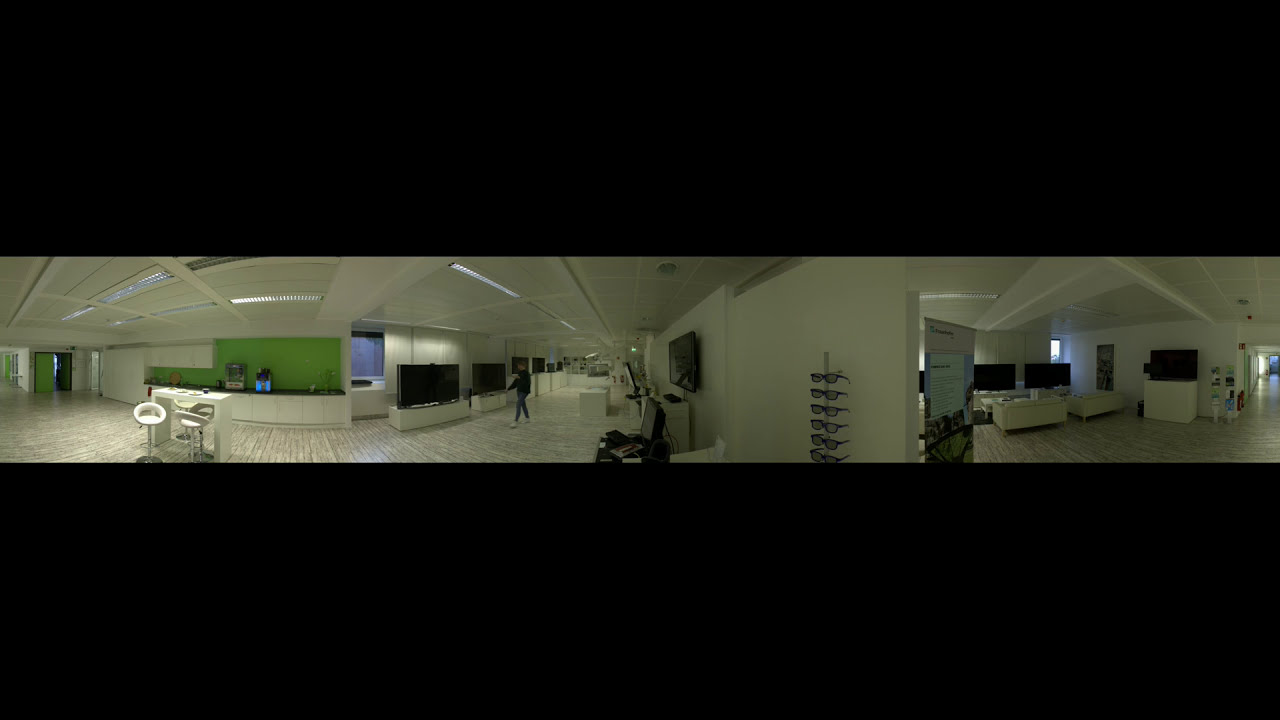The image is a 360-degree panorama of a modern office building, slightly distorted due to its wide-angle view. At the center of the scene, there's a kitchenette featuring a green backdrop and white cabinets, complemented by sinks and coffee makers. A light brown wooden floor extends through the space, harmonizing with the white ceiling adorned with long, narrow, rectangular lights. In front of the kitchenette, a white, rectangular-shaped table with curved bar stools is arranged neatly.

Adjacent to the kitchenette, a portion of the space resembles a gallery with numerous black screen-like objects, possibly TVs, situated atop small white rectangular stands. Further into the corridor, more of these black screens are either hung on the walls or placed on stands, creating a continuous display on both sides. A single person, donned in a black shirt and jeans, can be seen walking through this corridor.

To the left of the image, there's a stand displaying a vertical row of sunglasses, reinforcing the possibility that this office could belong to an optometrist or a similar establishment. On the far right side of the image, two squared, low couches are arranged with a freestanding poster nearby. Behind the couches, there is a window which brings natural light into the white-walled space. The image captures a blend of functional areas—kitchenette, gallery, and a lounge—all within the confines of a sleek, professional office environment.